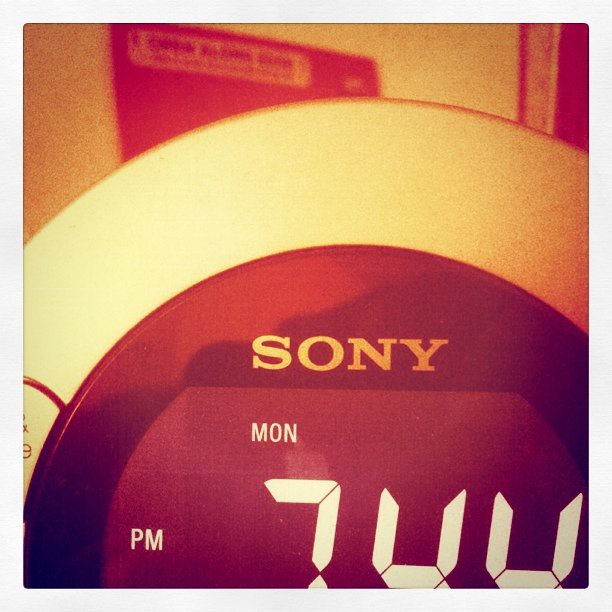This is a close-up photograph of a circular-shaped Sony device, likely an alarm clock, displaying the time and date on a black digital screen. The screen reads 7:44 PM and Monday. Encircling the black screen is a white circular border with metallic silver trim. The partially visible device bears the "Sony" brand name in white text at the top. The photo has an orange-yellow filter, adding a sepia-like hue to the image. The background appears grainy and unclear, revealing a white wall and a partially visible white doorframe. There are faint reflections on the clock's screen, hinting at the photo being taken with an iPhone, as some details suggest an Apple logo reflection.